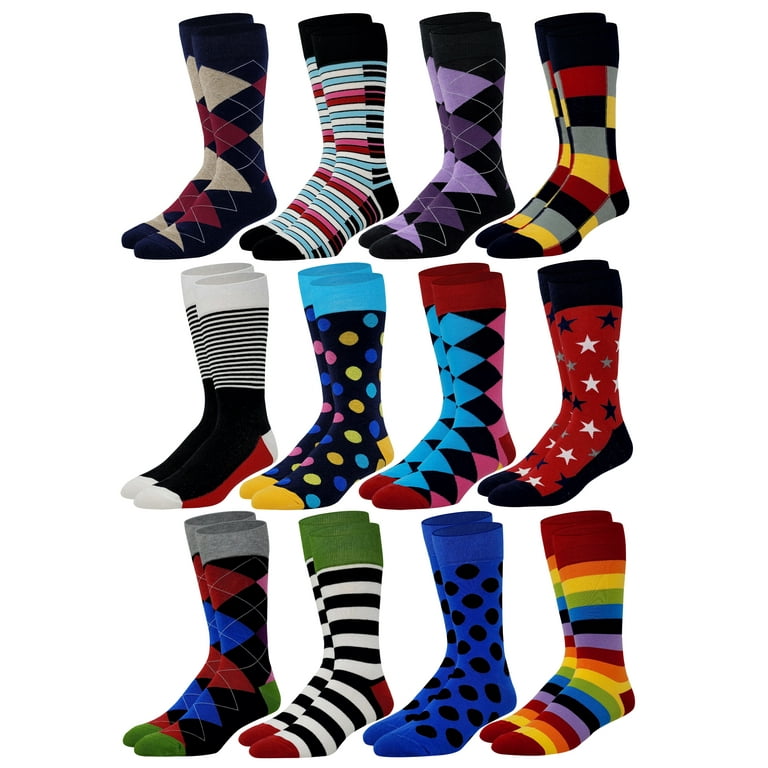This image showcases an array of 12 pairs of socks meticulously arranged in a grid format, evenly spaced and displayed from a side view with toes facing left. Organized in three rows of four pairs, each sock features a unique and vivid design. The top-left pair sports a white and pink diamond (argyle) pattern, followed by a pair with a vibrant piano keyboard design in light blue, white, and fuchsia. Next, a pair with lavender and dark purple argyle patterns sits beside a checkered pair with red, blue, yellow, and black squares.

In the middle row, from left to right, the first pair exhibits bold black stripes on a red background, transitioning to solid black with a white toe. Adjacent is a pair adorned with multi-colored polka dots—yellow, blue, green, and pink—with a yellow toe and blue top. The following pair displays blue and pink triangles on a black background, featuring a red toe and top section. The final pair in the row boasts a red background adorned with black and white stars, complemented by a black toe and top.

The bottom row starts with a classic black, red, and blue argyle pattern complemented by gray tops and green toes. Next is a pair of blue and white striped socks with a red heel and toe, finished with a green top. This is followed by a solid royal blue pair featuring black dots. The last pair is striking with rainbow stripes and red toes, rounding out this visually engaging and detailed display of diverse sock styles.